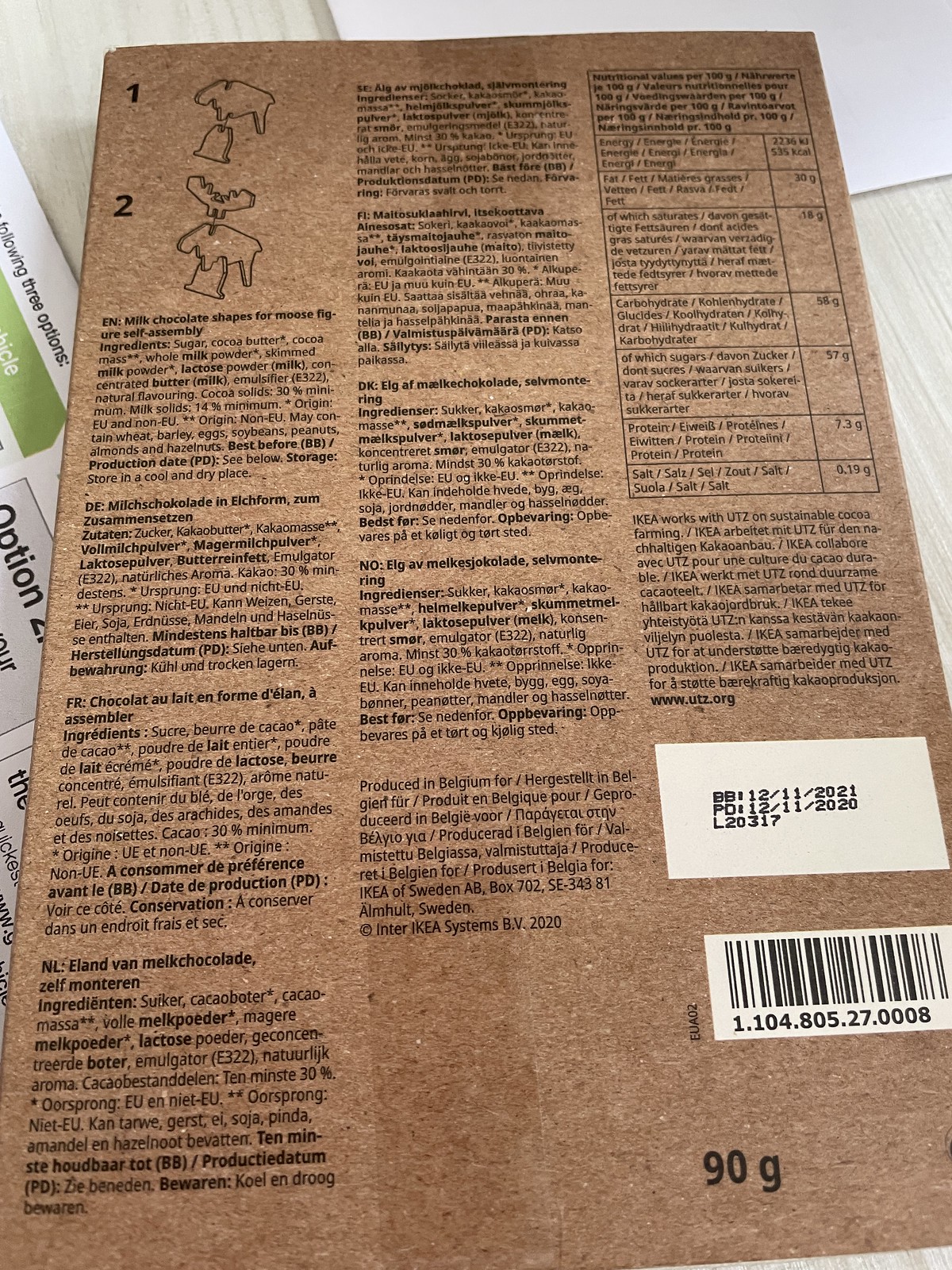The image features a brown, textured, flat object that closely resembles an envelope or package. This object is rectangular and appears similar to a book. It is prominently covered in black writing, which provides information about its contents and purpose. 

In the top left corner, there are black illustrations marked with the numbers 1 and 2, depicting the assembly process of a moose cutout. The assembly consists of three interlocking pieces: a base, a moose body, and moose ears. 

The text indicates that the object is a self-assembly kit for a moose figure made entirely of milk chocolate, adding a playful and edible twist to the typical assembly kit. Detailed information about the chocolate product is also present on the surface.

The package rests on a light-colored background, possibly a table or counter, and it is partially overlapping several other items, such as white papers or additional envelopes.